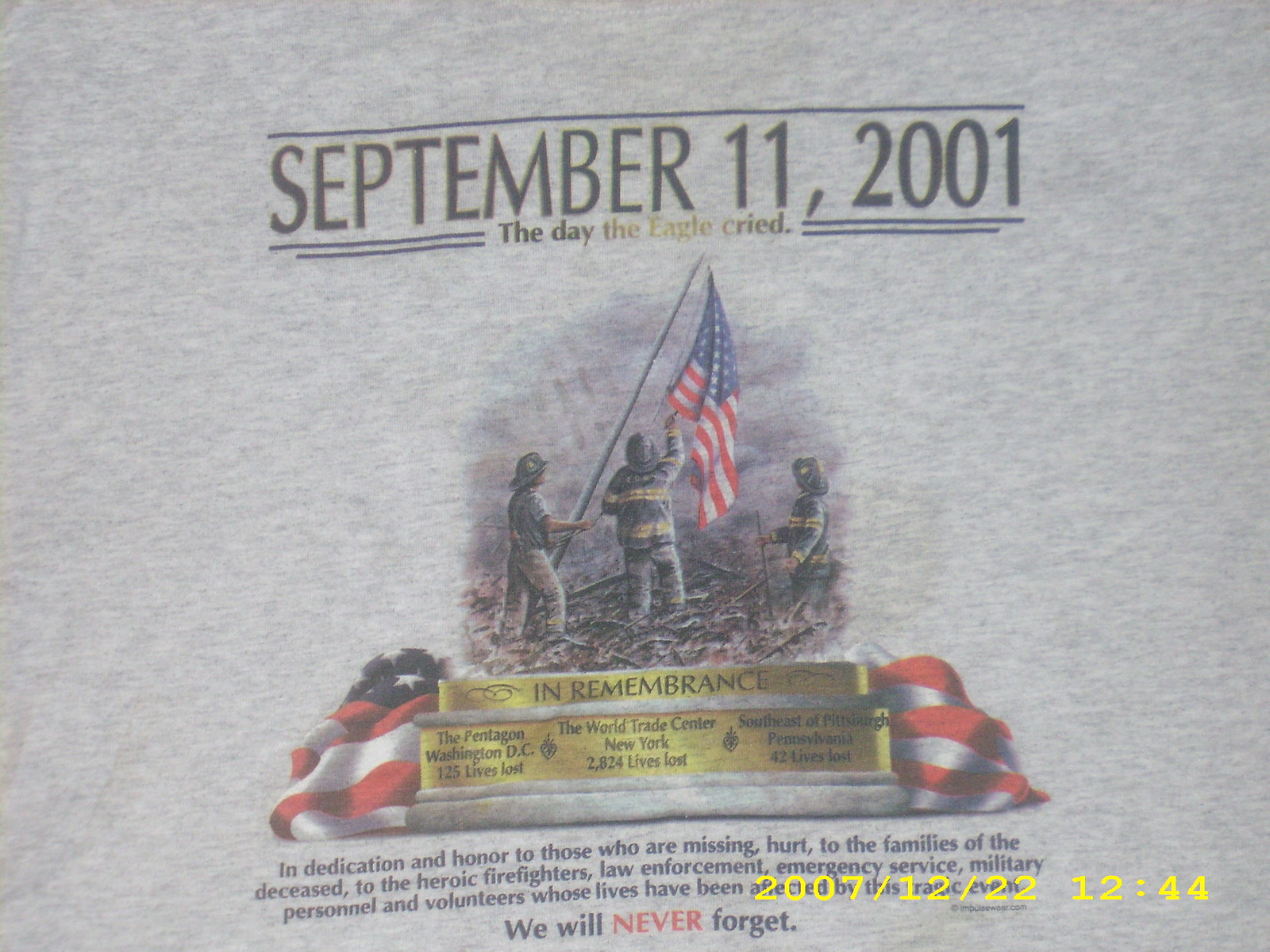The image depicts a commemorative poster on a textured, handmade-looking paper with a white and grayish background. At the top, it prominently displays the title "September 11, 2001" in large letters, followed by the subtitle "The Day the Eagle Cried" in smaller text. Central to the image is a poignant photograph of three firefighters hoisting an American flag amidst the rubble, reminiscent of the iconic Iwo Jima photo. Below the photo, a section marked "In Remembrance" lists the tragic losses: "The Pentagon, Washington, D.C., 125 lives lost; The World Trade Center, New York, 2,824 lives lost; Southeast of Pittsburgh, Pennsylvania, 42 lives lost." Another American flag subtly forms the backdrop of this information. At the bottom, the text honors the affected individuals: "In Dedication and Honor to Those Who Are Missing or Hurt, to the Families of the Deceased, to the Heroic Firefighters, Law Enforcement, Emergency Service, Military Personnel, and Volunteers Whose Lives Have Been Affected by This Tragic Event," concluding with the solemn declaration, "We Will Never Forget." The poster includes a copyright mark from ImpulseWear.com and a timestamp in yellow reading "2007-12-22 12:24 a.m." in the bottom right corner.